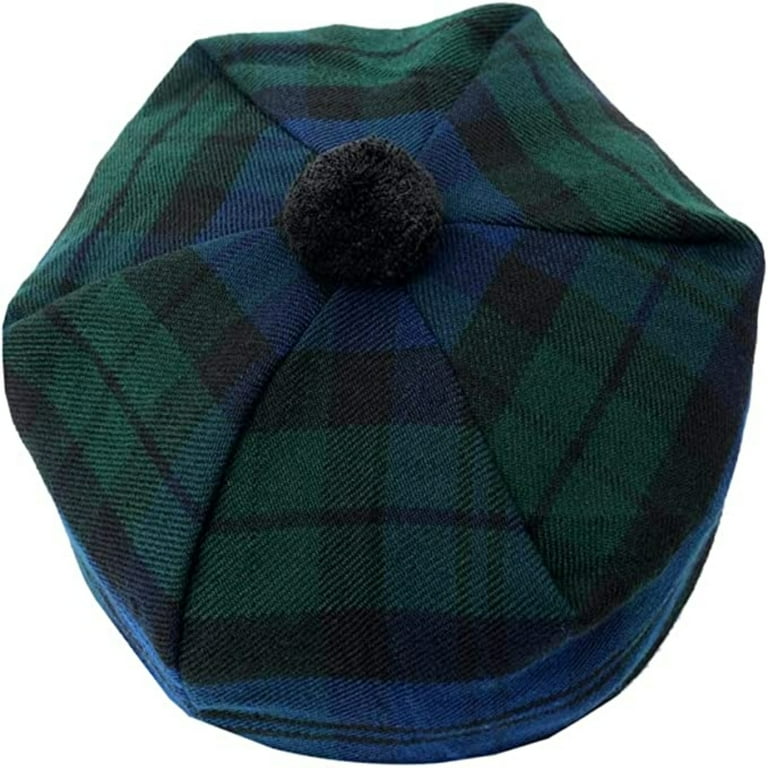This image features a modern yet vintage-inspired driving cap reminiscent of 1920s golfing attire, often worn by Scotsmen and commonly seen in sporting events. The cap is made from a tartan fabric, combining dark blue, jeans blue, light blue, forest green, and touches of black in a plaid pattern, creating a stylish yet classic look. The hat is stitched rather than knitted, and it includes a small black pom-pom at the center top. The fabric is folded beneath the pom-pom, giving it a gathered appearance. Unlike typical driving caps or kangol hats, this one is visor-less, maintaining an equal brim around all sides, ensuring it covers the head uniformly. This cap is not merely a yarmulke but a trendy headpiece to be perched lightly atop the head, serving more as a fashion accessory that keeps the scalp warm rather than shading the eyes.